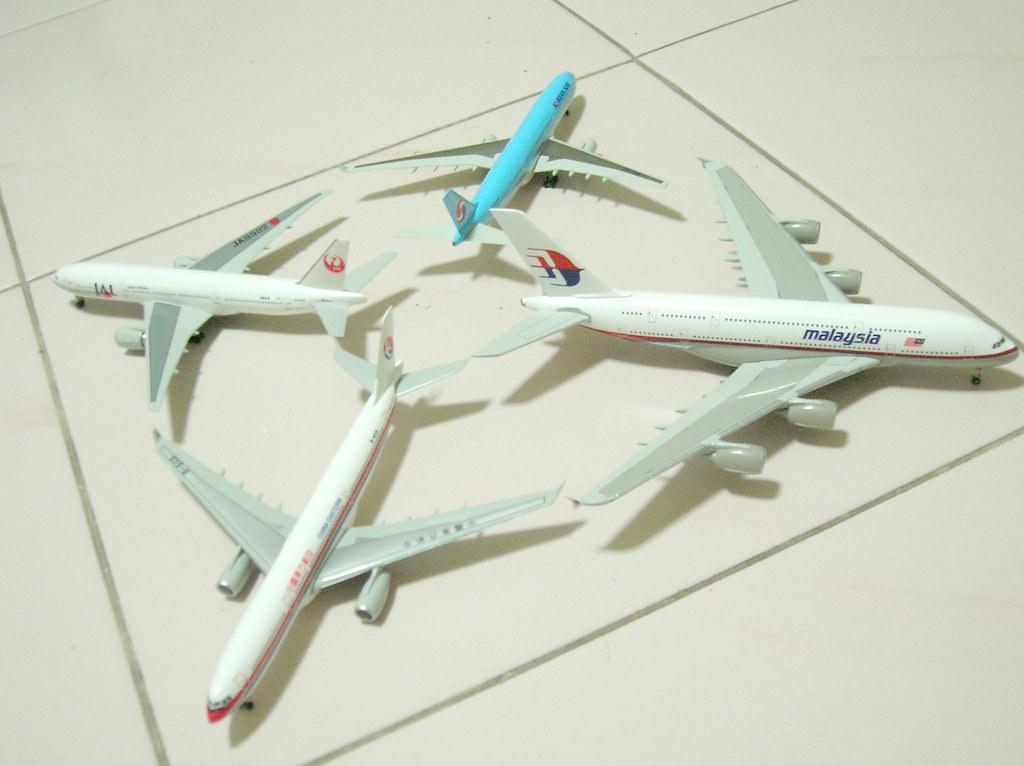This color photograph features four miniature toy airliners, arranged with their tail fins touching at the center, forming a cross pattern. The airliners are positioned so that each nose points outward toward the corners of a single white tile, perfectly fitting within its bounds. The floor is comprised of large white tiles with gray grout between them.

The airliners vary in appearance and size, though all are roughly scaled to occupy the space of one tile. Three of the planes are predominantly white with gray wings, one of which prominently displays the word "Malaysia" on its fuselage along with a red and blue logo on its tail fin. The fourth airliner, distinguished by its blue coloration and gray wings, faces the top of the photograph and features a red, white, and blue circular logo on its tail.

Additional details include small amounts of unreadable writing on the other planes, a red nose on the plane closest to the observer, and a small dot on the tile beneath it. The arrangement creates a visually appealing pattern that highlights the careful placement and design of these model jets.